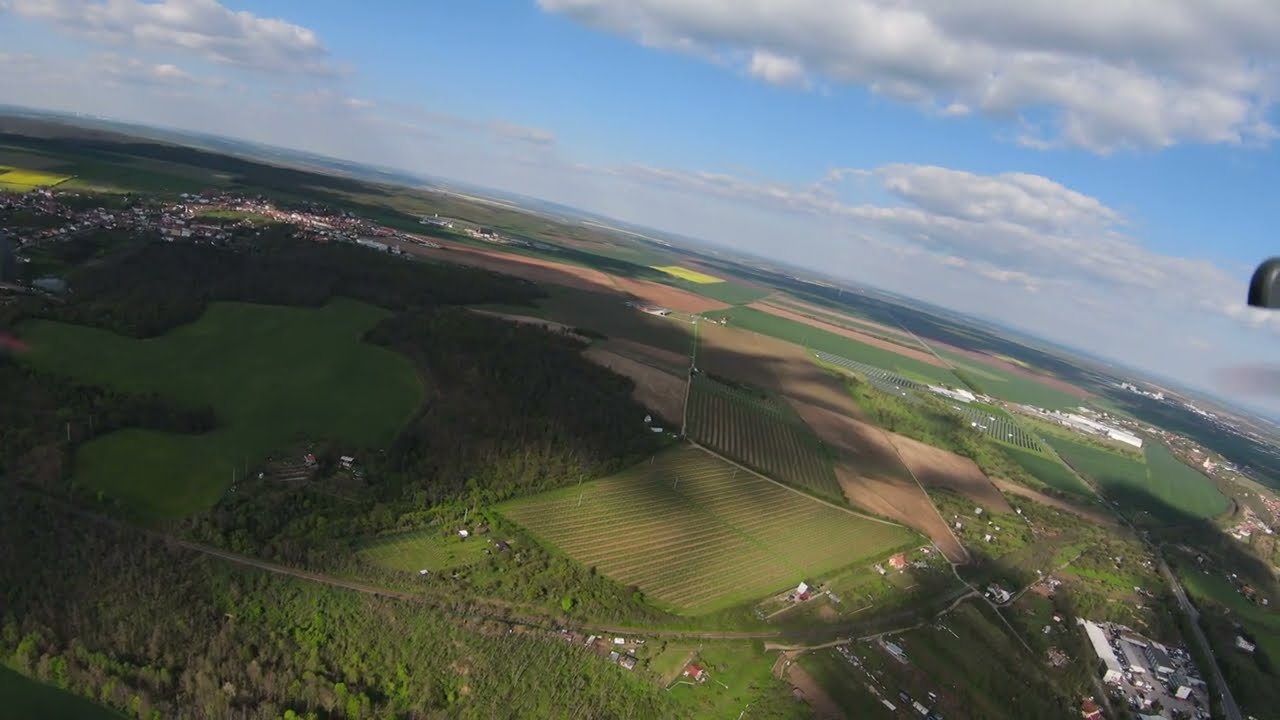The image is an aerial photograph taken at a high altitude, likely from an airplane, capturing a vast rural area with lots of farmland and small towns. The landscape below is predominantly flat, possibly indicating a prairie region. The dominant feature in the image is an extensive patchwork of farm fields, varying in colors from greys and light browns to dark browns and yellows, arranged in a grid-like pattern. Scattered amongst these fields are clusters of woodland areas and a body of water surrounded by trees.

In the top left corner of the image, a small town is visible, characterized by numerous white and brown buildings arranged along a network of roads. This town forms a dense community in contrast to the more spread-out farmhouses seen elsewhere in the image. Moving to the bottom left, there's a well-cultivated area with curves and arches that could be reminiscent of a golf course, enveloped by woodland. 

The sky, dotted with clouds, casts shadows on different parts of the landscape below. The left side of the image is more shaded due to cloud cover, whereas the right side is bathed in sunlight, accentuating the fields and buildings. There are visible dirt tracks and small roadways crisscrossing the scene, and a larger site or factory is noticeable in the bottom right-hand corner, adding an industrial element to the predominantly agricultural landscape. The image showcases a serene and orderly rural environment, interrupted only by the natural and man-made landmarks that dot the terrain.